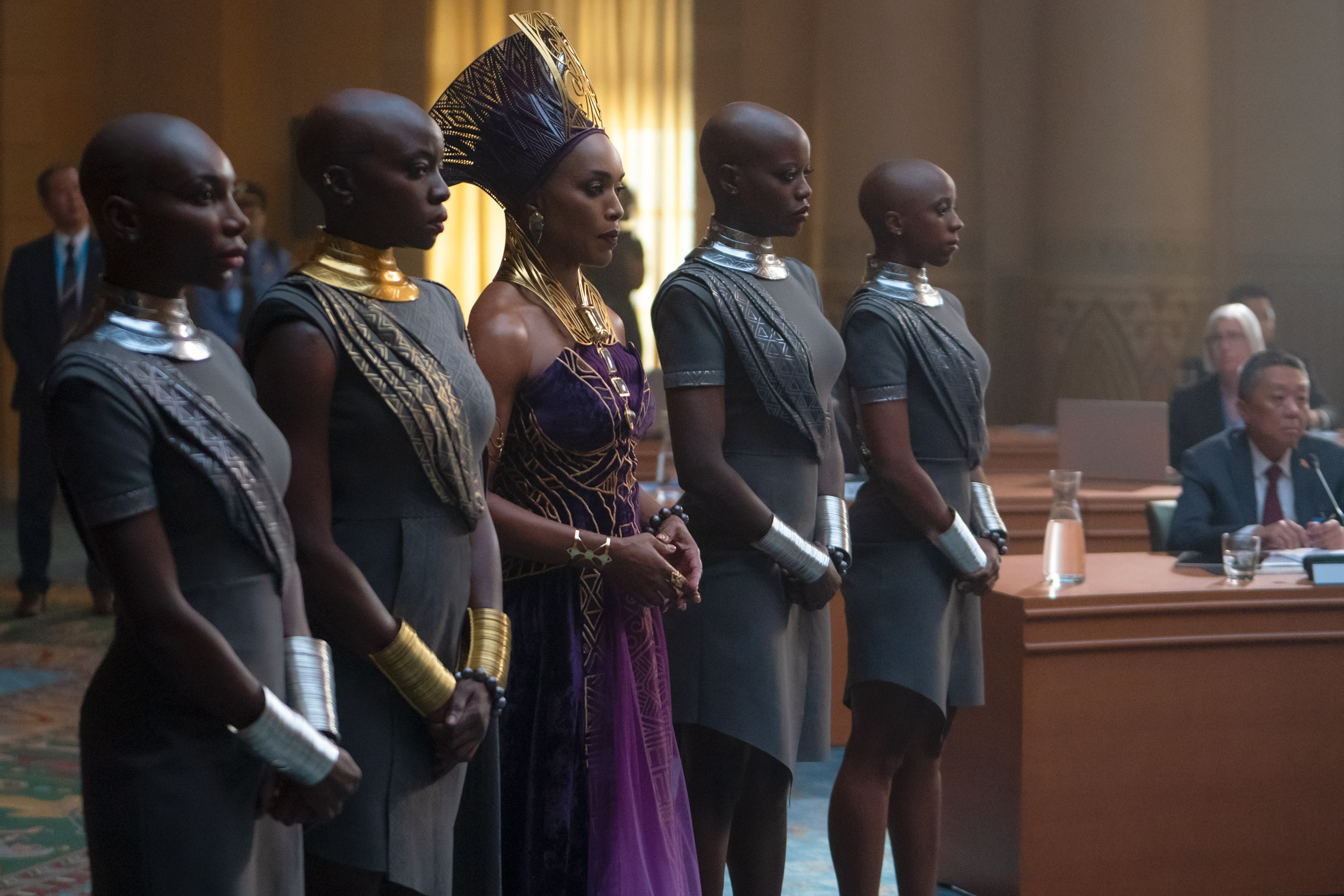In this detailed image set in a courtroom, five women stand prominently in the foreground. Four of them are Wakandan warriors from the Dora Milaje, identifiable by their bald heads and matching grey uniforms. Three of these warriors are adorned with silver bracelets and necklaces, while one distinguishes herself with gold jewelry. The fifth woman, standing centrally and distinctively, is dressed in an elegant purple dress accessorized with a matching headpiece, underlining her status as the Queen. The setting is confirmed by various courtroom elements visible in the background, where attendees include an old Asian man and an elderly white woman seated at desks. These desks also bear practical items like a laptop, a water jug, and a glass of water, further grounding the scene in a courtroom environment. The Dora Milaje stand protectively around the Queen, who exudes regal authority, while all five women gaze steadfastly in the same direction.